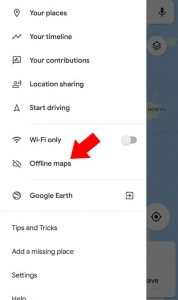The image depicts a screen interface, likely from a mobile application related to navigation or location tracking. Visible beneath a series of translucent menu options is a grayed-out digital map. Prominently featured is an icon that resembles a settings cog, suggesting the menu is for configuration purposes. The menu options include "Your Places," "Your Timeline," "Your Contributions," "Location Sharing," "Start Driving," "Wi-Fi Only," "Offline Maps," "Google Earth," "Tips and Tricks," "Add a Missing Place," and "Settings." Towards the bottom of the menu, the word "Halo" (or possibly "Helo," though it is partially cut off) appears. A large red arrow points to the "Offline Maps" option, and notably, the "Wi-Fi Only" toggle is not activated. The layout and features are reminiscent of family driving or tracking apps like Life360, though it is clearly not Life360 itself.